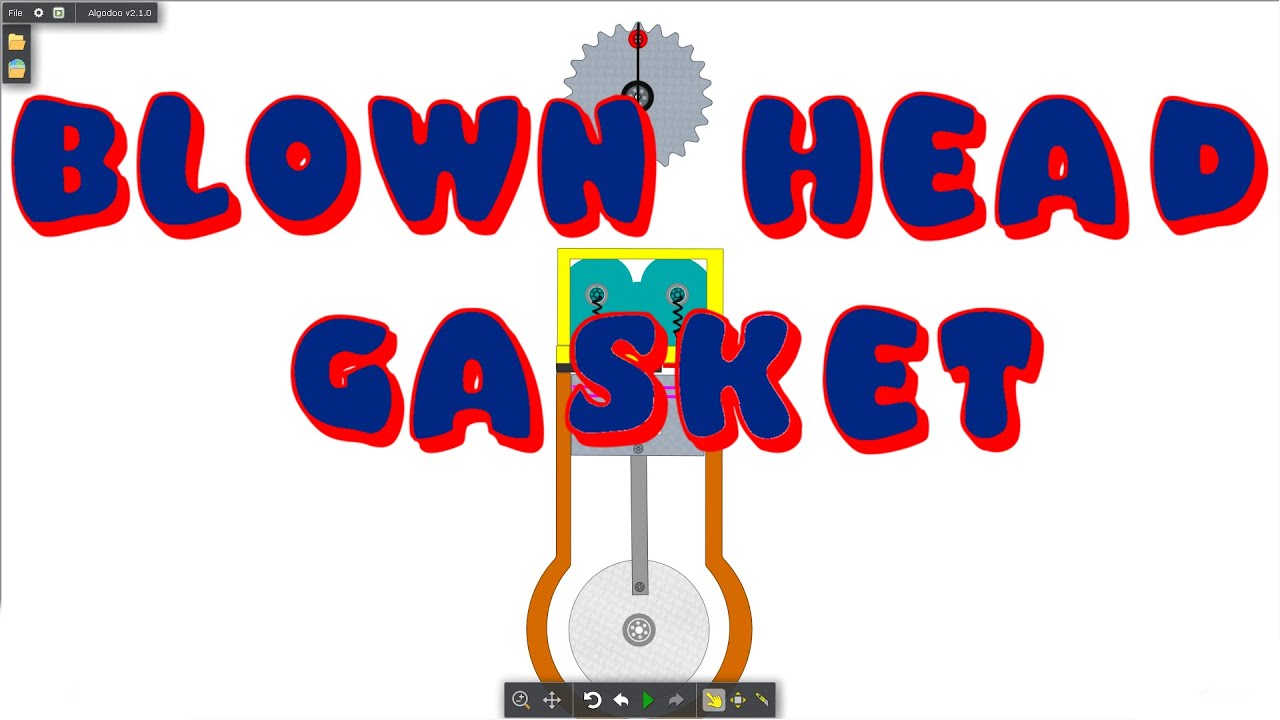The image presents an animated or diagrammatic representation of a blown head gasket, with "blown head gasket" prominently displayed in the center of the white background. The text is large, with a striking blue font at the core and a glowing red border. At the top center, a gray circular rotary disc or cutting blade is depicted. Below this, there is a piston-like figure with a gray wheel at the bottom, connected to a shaft of the same color. This assembly is encased in a yellow frame, with a yellow rectangle at the top attached to a green coiled spring.

The top left corner of the image features L-shaped icons set against a black background, resembling control panel or interface tools, similar to those found in applications like Photoshop. Another set of buttons or interface tools is located at the bottom of the image, also against a black background. Additionally, there is a detailed depiction of a red circle with the number six inside it, located below what appears to be a gear.

In summary, the image is intricately styled as an illustration within a digital application or browser window, highlighting the various mechanical components and control tools associated with the problem of a blown head gasket.